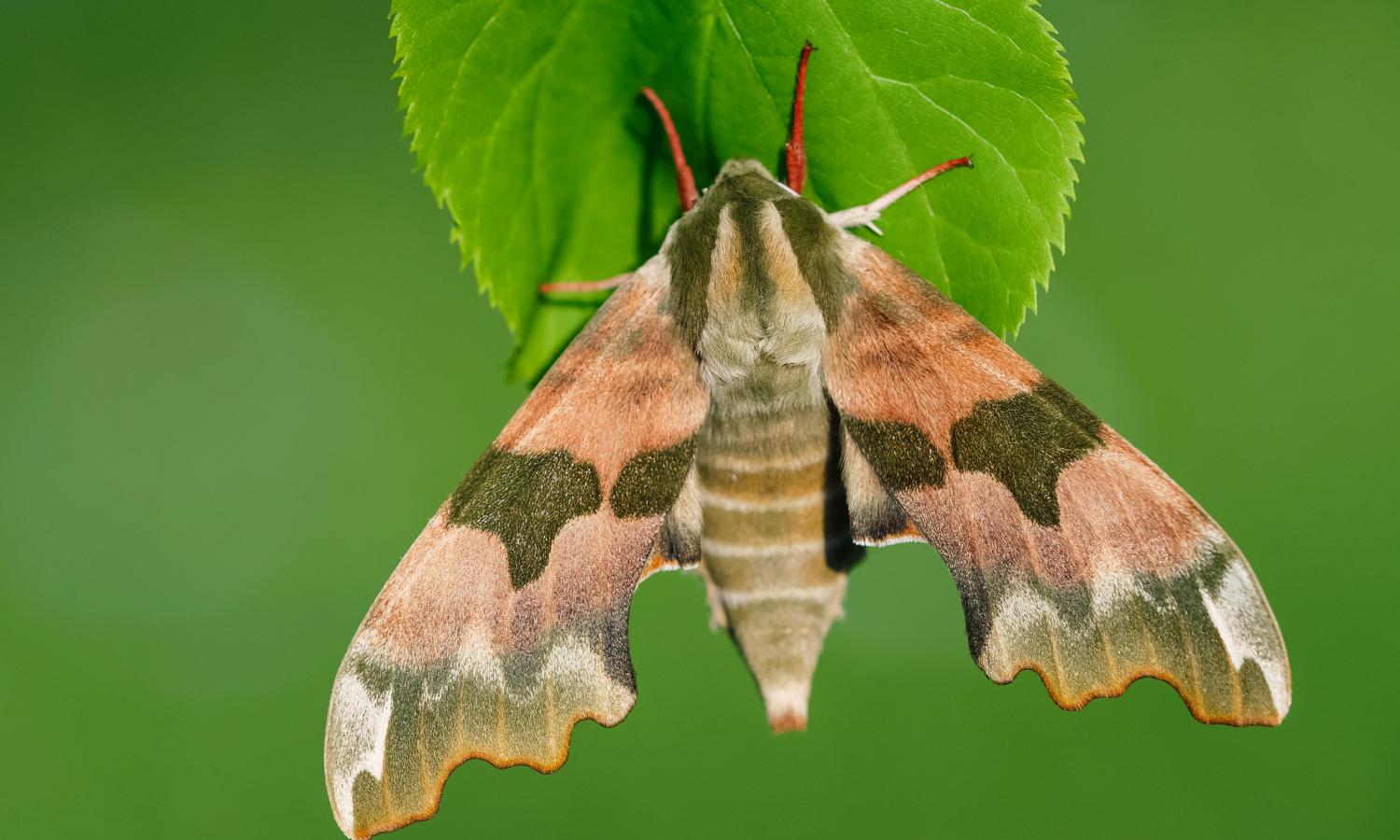This close-up photograph features a vividly colored moth resting on a green leaf that spans the top portion of the image. The moth's head is oriented towards the top of the photograph, showing off a mix of brown and green hues, adorned with two pairs of antennae: one white and one red. The body of the moth, showcasing tan and green shades with white stripes, extends downward, ending in a tail section that combines grayish and brownish-green tones with white accents.

The moth's wings are spread open, displaying an intricate pattern of colors. Starting near the head, the wings exhibit a blend of brown and orange, progressing to darker, blackish hues. Further down, lighter shades of gray, white, and then a combination of green and orange at the tips are visible. The contrasting colors of the moth's legs—red and white—add to its striking appearance.

The green leaf on which the moth rests also plays a significant role in the composition. The leaf emerges from both the top left and top right corners, partially obscured by the moth, and converges towards the center of the image. The background is a uniform green, devoid of discernible details, which helps to emphasize the intricate details and vivid colors of the moth.